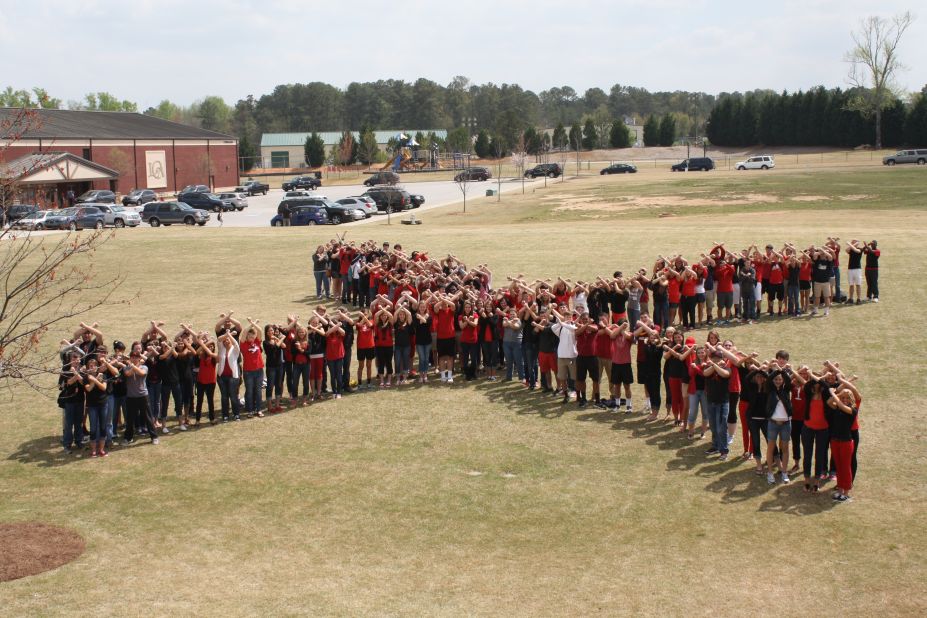This aerial photograph captures a vibrant scene outside what appears to be a school, identifiable by the playground with a red structure and a sloping gray roof situated to the left. In the foreground, approximately 100 to 150 students are arranged in the shape of a giant 'X,' forming two intersecting lines. Most are wearing red shirts and black pants, with a few in white, adding a striking visual contrast against the green and yellow dusty grass of the field. Each student has their arms raised above their heads or crossed in front of them in an 'X' pattern, facing the camera with big smiles. The image showcases a bright, light blue sky at the top, transitioning into a row of green trees lining the background. Below the trees, there's a parking lot filled with numerous gray and blue cars, which further emphasizes the scholastic setting. The central focus remains the joyful students creating a powerful, unified 'X' amid the sprawling landscape.